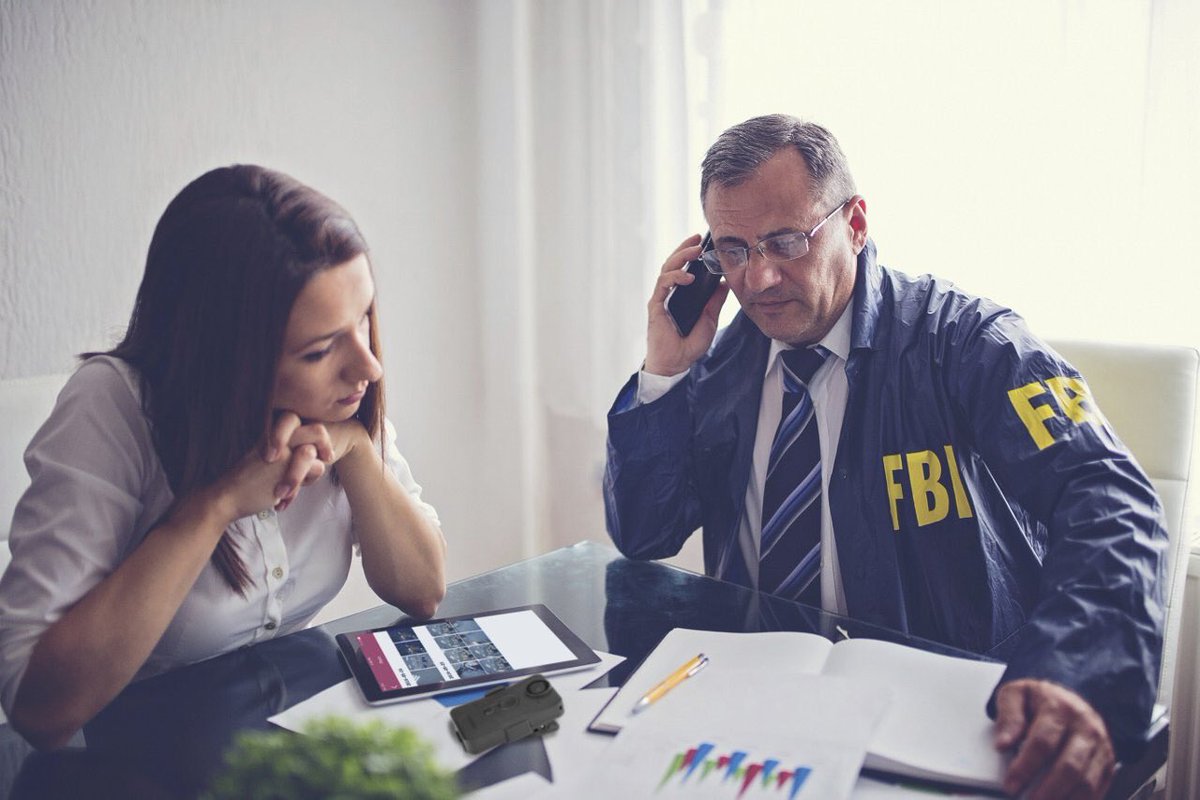This detailed photograph captures a scene in the center of an indoor setting, likely a kitchen, with a solid white wall and a white curtain in the background. Two individuals are seated at a table approximately in the middle of the image. The man on the right is wearing an FBI jacket with bold letters identifying his affiliation with the Federal Bureau of Investigation on both the front and his left arm. He is engaged in a phone conversation and wears glasses. In front of him are various items on the table, including an open book, a pencil, and a chart that both he and the woman are examining. The woman, seated to his left, has brunette hair and is dressed in a long-sleeve button-up shirt. Next to her lies an iPad, adding to the assortment of materials on the table. Their body language suggests they are collaborating on some investigative work, with no indication of an adversarial relationship. The overall palette of the scene includes tones of white, off-white, brown, green, red, blue, and yellow, indicating a predominantly neutral and soft color scheme. The image captures a moment of focused teamwork within a domestic, daytime environment.